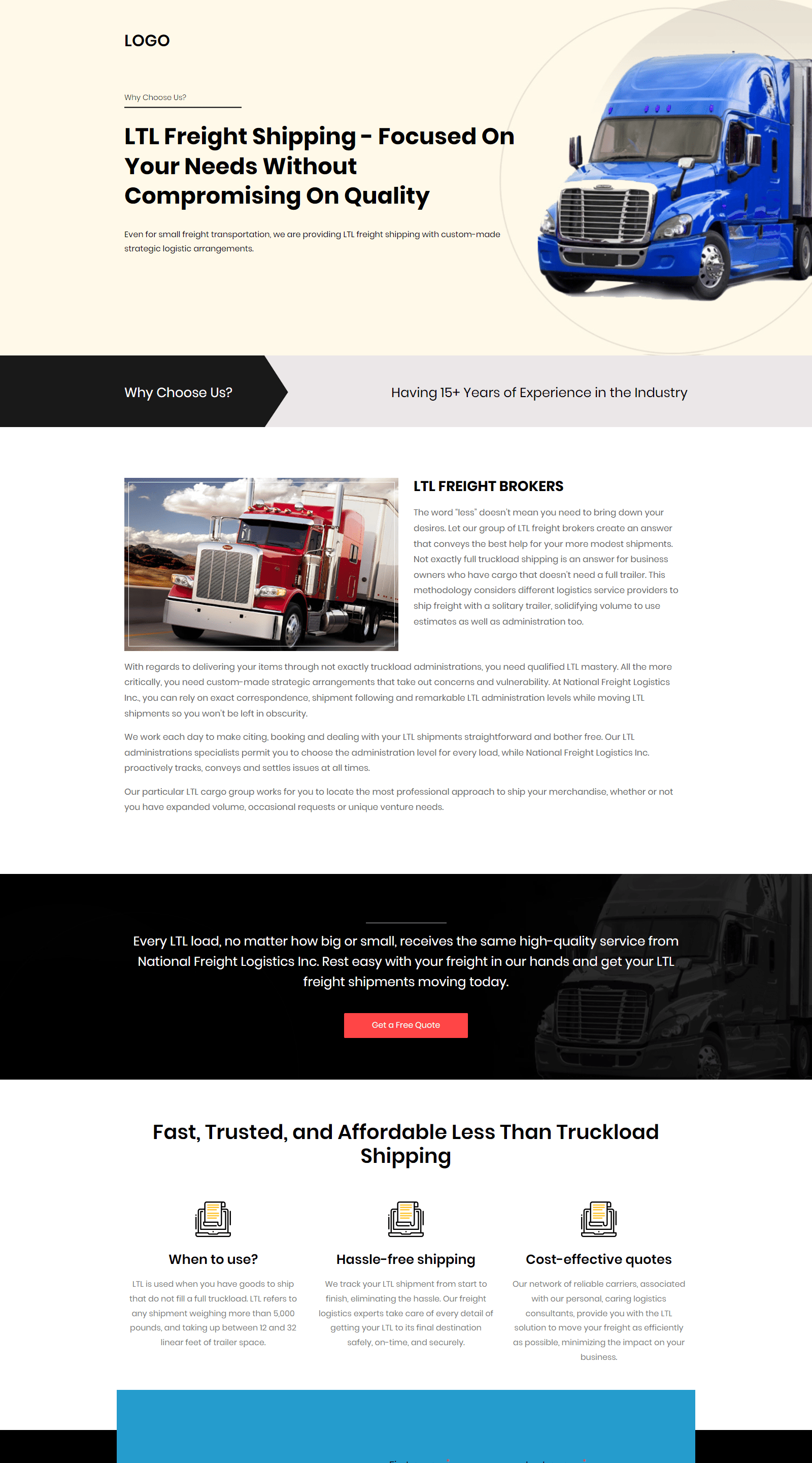The website features a professionally designed layout with a prominent logo positioned on the top left-hand corner of the banner. The main visual element is a large image of a blue semi-truck, viewed from the front, with its hood and front wheels visible. The truck is angled slightly towards the lower left side, emerging from the right side of the image.

Adjacent to the truck image, towards the left, is a light yellow banner with bold text that reads, "LTL Free Shipping: Focused on Your Needs Without Compromising on Quality." 

Beneath this is a thinner banner divided into two sections. The left section is black with white text that asks, "Why Choose Us?" The adjacent portion is grey and states, "Having 15+ years of experience in the industry."

At the bottom of the layout, there is another slender section featuring a blurb accompanied by an image of a tractor-trailer, marking the beginning of a descriptive paragraph.